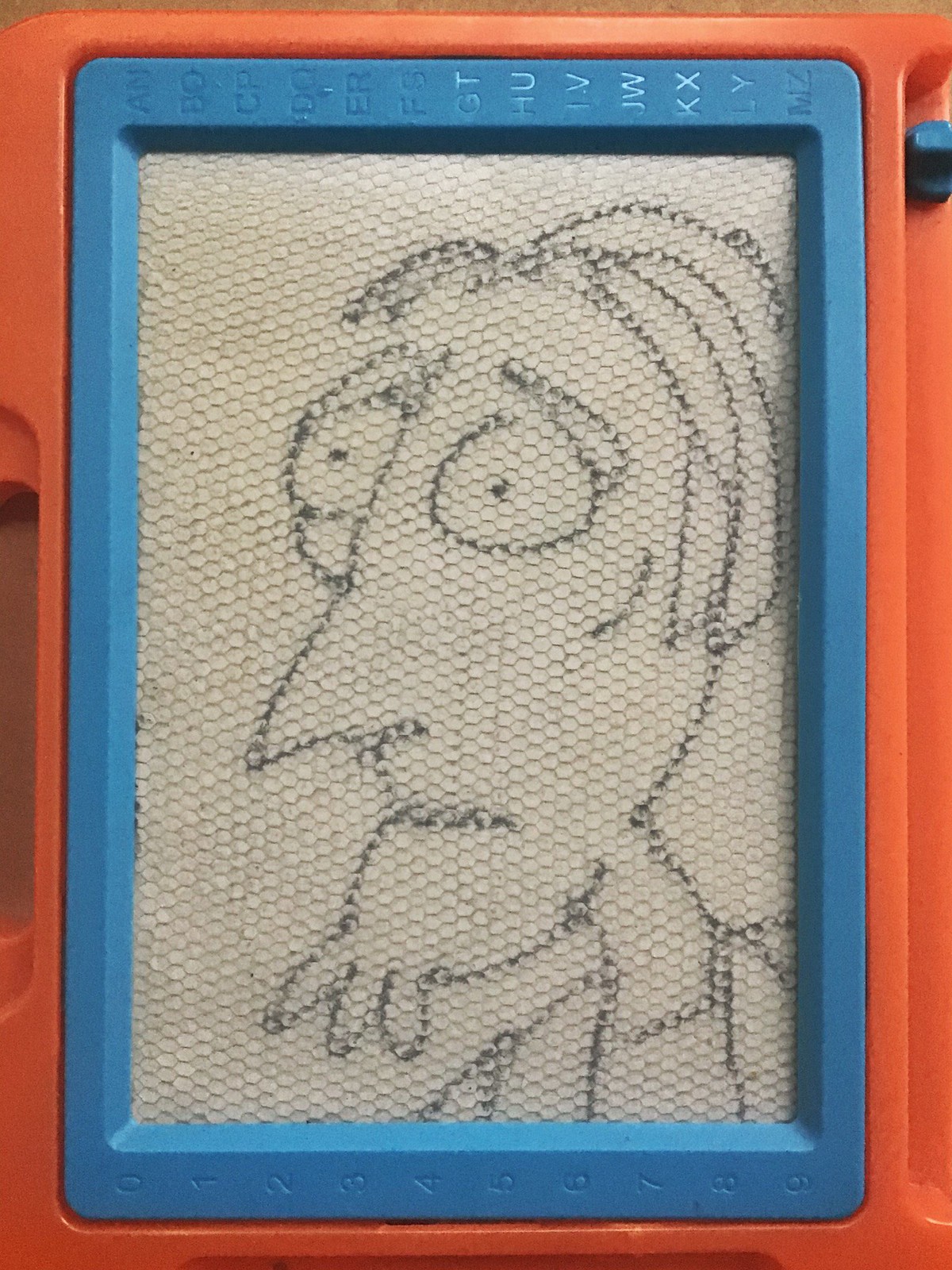In this detailed photograph, we observe a classic children's magnetic drawing toy featuring a grey screen. Utilizing a magnetic pen, users can manipulate small magnetic particles beneath the surface to create illustrations. In this particular instance, the drawing on the screen depicts a man with distinct features. He has a very pointed nose, bulging round eyes adorned with eyebrows, and short, uniformly-length hair. His facial hair includes a neatly drawn goatee. The man’s expression appears somewhat apprehensive, as conveyed by the artist’s careful rendering of his mouth. Additionally, his neck and the top of his shirt are visible in the drawing, completing the character’s depiction on this nostalgic toy.